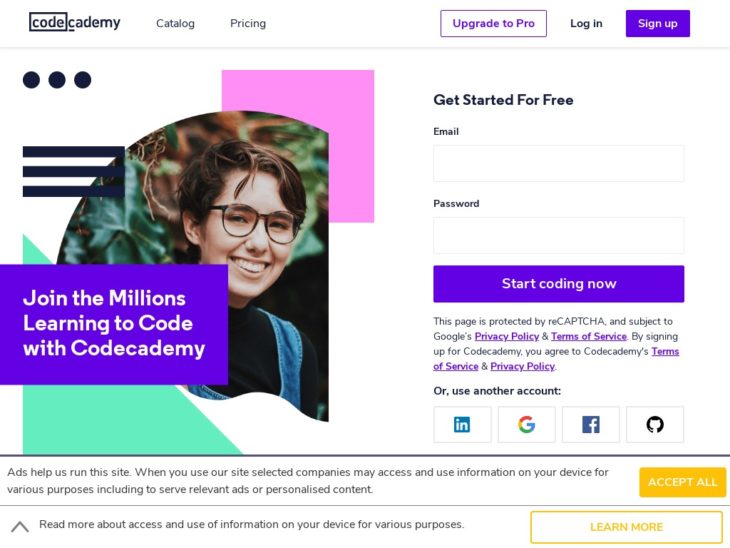This horizontal image, captured from a webpage accessible via computer or smart device, showcases the homepage of Code Academy against a stark white background typical of a computer screen. 

In the upper-left corner, the logo "Code Academy" appears, with "Code" highlighted by a box around it. Adjacent to this are navigation options: "Catalog" and "Pricing". On the upper-right side, several interactive elements include "Upgrade to Pro" in a purple boxed text, a "Login" option in black, and "Sign Up" in purple.

Below this header, a gray line demarcates the subsequent section. Prominently displayed are three large horizontal circles, each accompanied by various geometric shapes. Dominating this section is a photograph of a young woman wearing glasses, smiling warmly into the camera. Above her, text reads: "Join the millions learning to code with Code Academy."

To the immediate right, a call-to-action invites users to "Get started for free." Below this, fields for email and password entry are provided, along with a purple button labeled "Start coding now." This area also mentions the site's protection by reCAPTCHA and links to privacy policies and terms of service.

Additional options allow users to register using social media accounts, indicated by clickable icons for each platform. Lastly, the page includes information about ads that support the site, offering users the choice to "Accept All" or "Learn More."